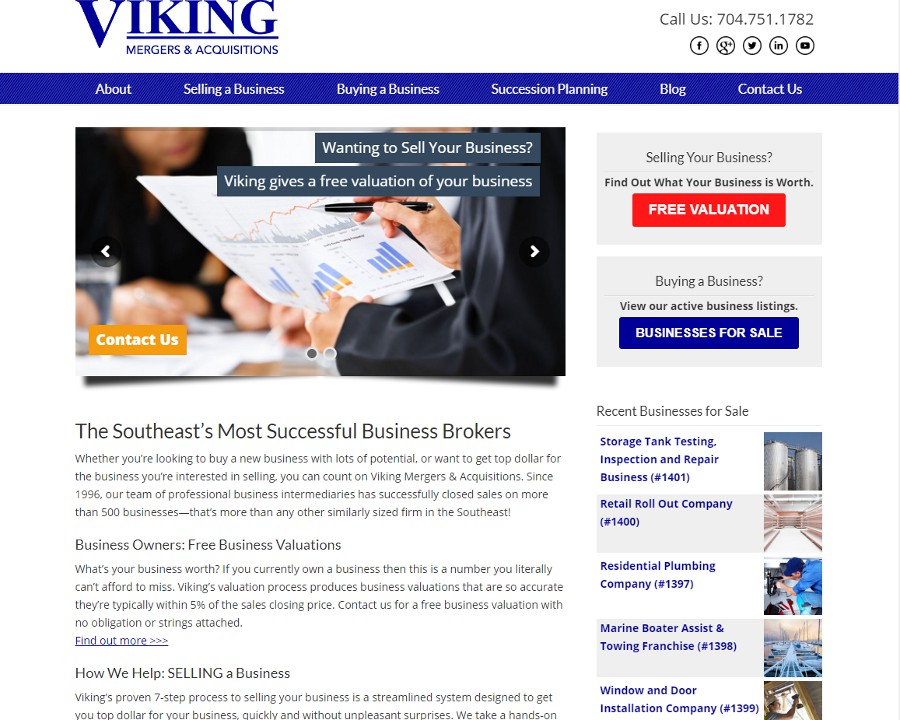The image depicts a well-organized website centered on biking-related mergers and acquisitions. The header features a white background with blue accents, prominently displaying the site’s name alongside the terms "Biking, Mergers, and Acquisitions." In the upper right corner, there's a "Call Us" prompt with a phone number, accompanied by social media icons linked to Facebook, Twitter, Instagram, and YouTube.

Below the header is a dark blue navigation bar offering various sections, including "About," "Selling a Business," "Buying a Business," "Succession Planning," "Blog," and "Contact Us." Below this, there is an image of a person holding a piece of paper displaying bar graphs. The text adjacent to the image reads, "Wanting to Sell Your Business? Biking gives you a free valuation of your business." A "Contact Us" button is positioned at the bottom left of this section.

Further down, the title "The Southeast’s Most Successful Business Brokers" introduces a detailed segment. On the far right, there is a section dedicated to "Selling Your Business" with a clickable red button for a free evaluation. Just below it, the "Buying a Business" section offers a blue "Businesses for Sale" button. A list of "Recent Businesses for Sale" follows, showcasing various opportunities such as a storage tank testing, inspection, and repair business; a retail rollout company; a residential plumbing company; a marine boat towing franchise; and a window and door installation company.